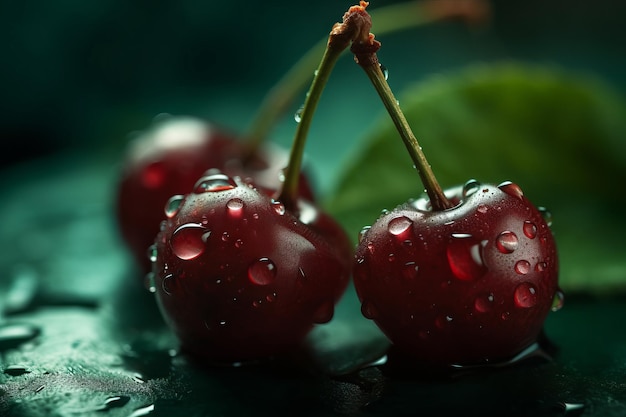The image is a detailed close-up photograph featuring three dark red cherries adorned with water droplets, likely from rain or being rinsed. The cherries are placed on a dark green, wet surface that resembles a large leaf. In the foreground, two cherries are in sharp focus, leaning slightly toward each other and touching at the top with their green stems still intact. Both cherries also display glistening water droplets. Directly behind these two, there is a third cherry, partially obscured and blurred due to the shallow depth of field employed in the photograph. This third cherry also has water droplets and a visible green stem. The background of the image is dark and blurred, adding a sense of gloom, with a prominent green leaf positioned on the right side, further enhancing the scene's naturalistic and wet ambiance.